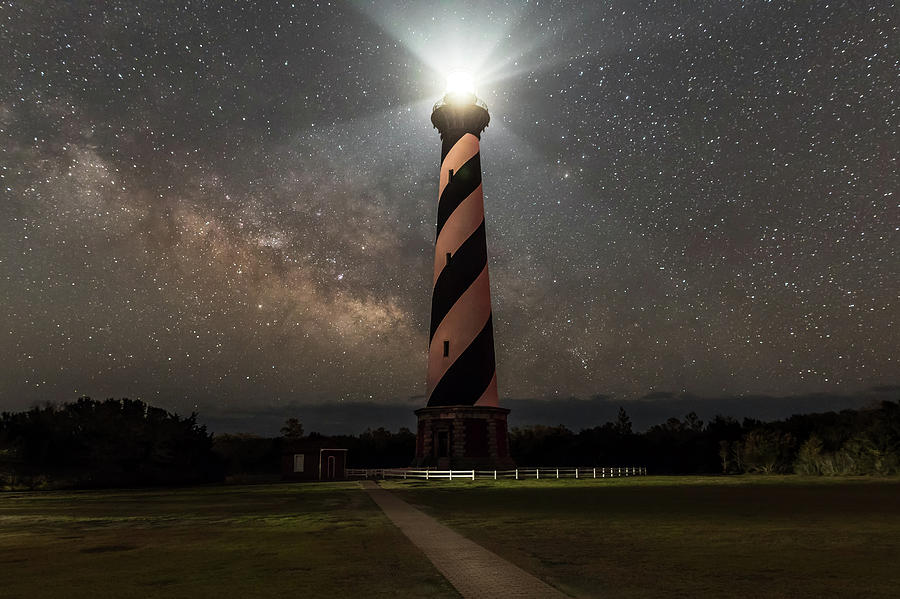This detailed 3D image depicts a striking black and yellow striped lighthouse prominently centered amidst a large field. A long, cemented pathway resembling a sidewalk stretches from the bottom middle of the image, traversing through the grass and leading directly to the lighthouse. The lighthouse features a white fence encircling its base, and at the tower's top, an intense bright light serves as a beacon, casting beams upward and outward, illuminating the scene. The surroundings are adorned with dark trees and distant mountains, all under a night sky speckled with stars and scattered clouds, contributing to a serene nocturnal ambiance. The sky is not completely black, allowing the lighthouse’s powerful illumination to highlight the environment, casting light on the ground and the fence.